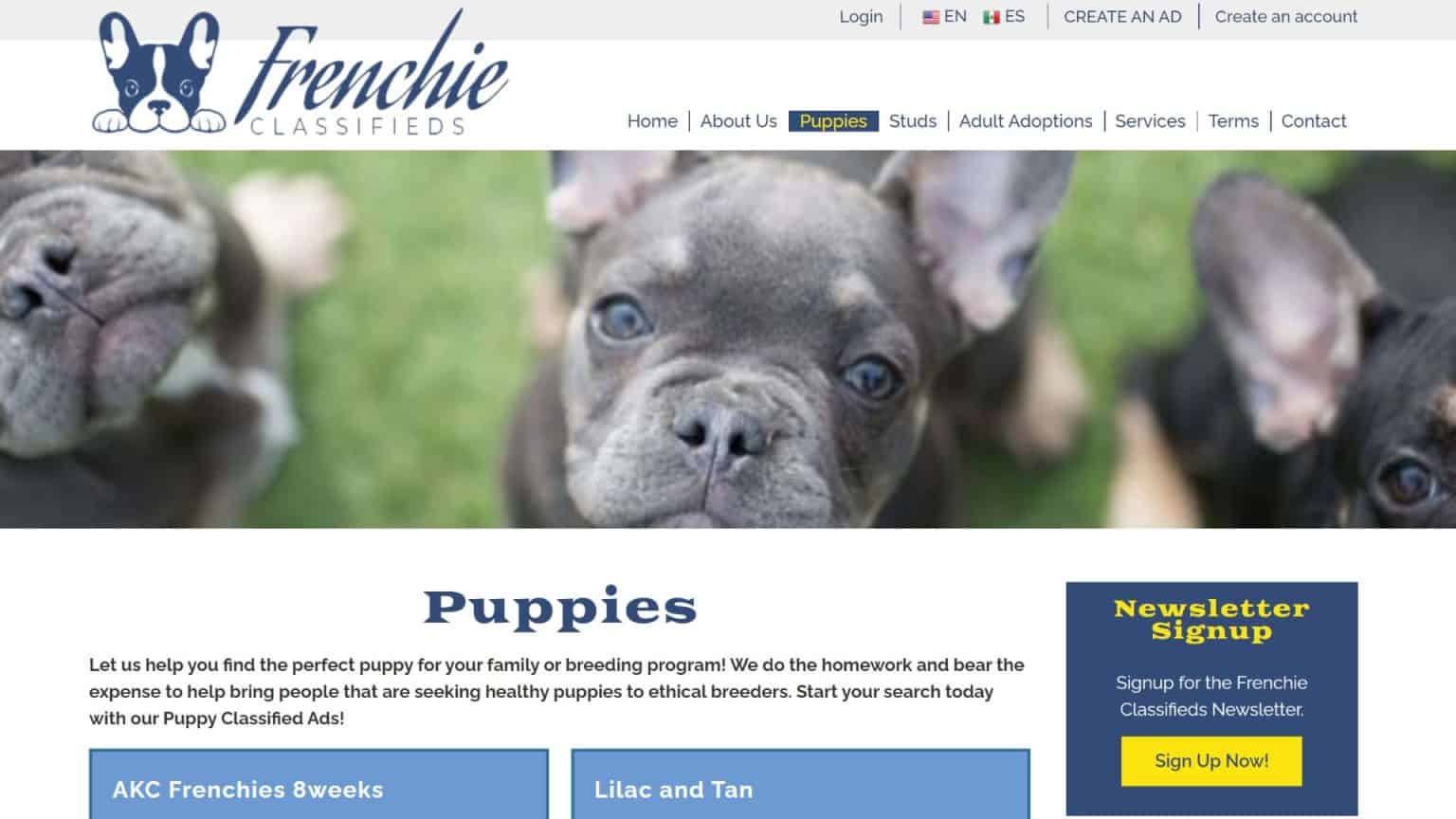The image is a rectangular newsletter layout dedicated to French Bulldogs. The page is oriented horizontally, with the longer sides stretching from left to right. A light gray border spans the middle of the page, featuring blue text that includes options such as "Log In," "EN or ES," "Create an Ad," and "Create an Account."

Below this border, a small picture of a blue and white French Bulldog is displayed, accompanied by the words "Frenchie Classifieds" in italicized font. Moving further down, a navigation menu is centered, listing tabs such as "Home," "About Us," "Puppies," "Studs," "Adult Adoptions," "Services," "Terms," and "Contract." The "Puppies" tab stands out, highlighted in dark blue with yellow letters.

Dominating the middle of the page, a horizontal image showcases three French Bulldogs, with the central one prominently in focus and gazing directly at the viewer. Beneath this image, a text section titled "Puppies" invites readers to find their perfect puppy for family or breeding purposes. The accompanying message emphasizes the organization's dedication to connecting prospective puppy owners with ethical breeders, mentioning their commitment to conducting thorough research and covering related expenses. The call to action encourages users to start their search through the puppy classified ads.